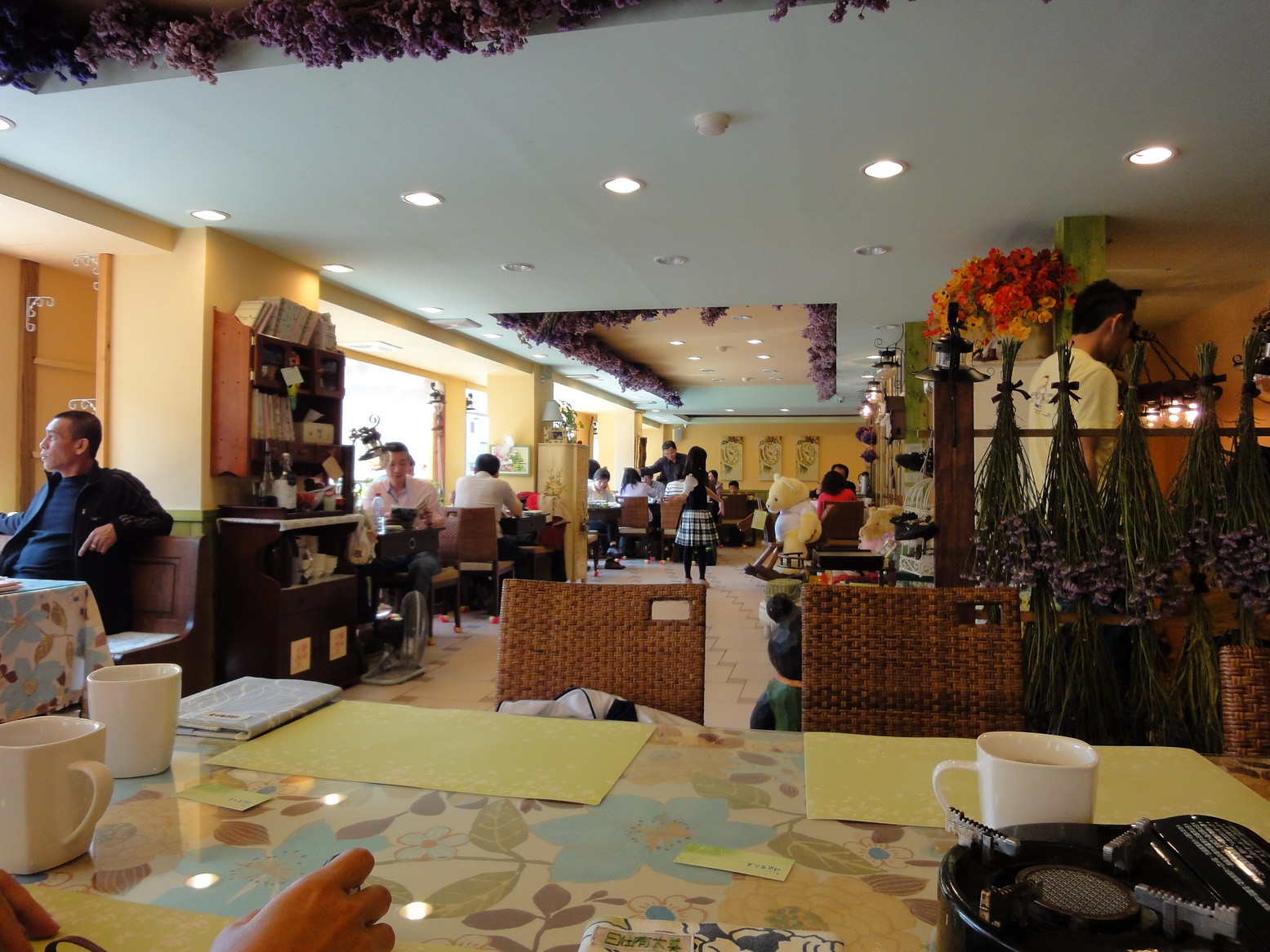The photograph captures the interior of a spacious restaurant, possibly situated in a hotel, bathed in daylight streaming through a large window on the left side, where a man in a long-sleeved blue shirt is leaning back and gazing outside. The floor is white, providing a clean contrast to the pale yellow walls and white ceiling adorned with hanging purple flowers, which are mirrored by matching floral decorations below. 

To the forefront, there's a table set with yellow placemats and surrounded by two brown bamboo-looking chairs, with three coffee mugs, one of which remains untouched. Adjacent to this, a table is partially occupied, with a jacket draped over an empty chair and a newspaper lying next to it. The restaurant layout includes an open central walkway, hinting at a buffet section on the right side. 

Towards the background, various other diners are seated, some against the wall lined with additional seating. Notably, a large yellow teddy bear and a woman standing before it add a whimsical touch to the setting. Additional decorations include flowers on the ground, reinforcing the restaurant's cozy yet vibrant atmosphere.